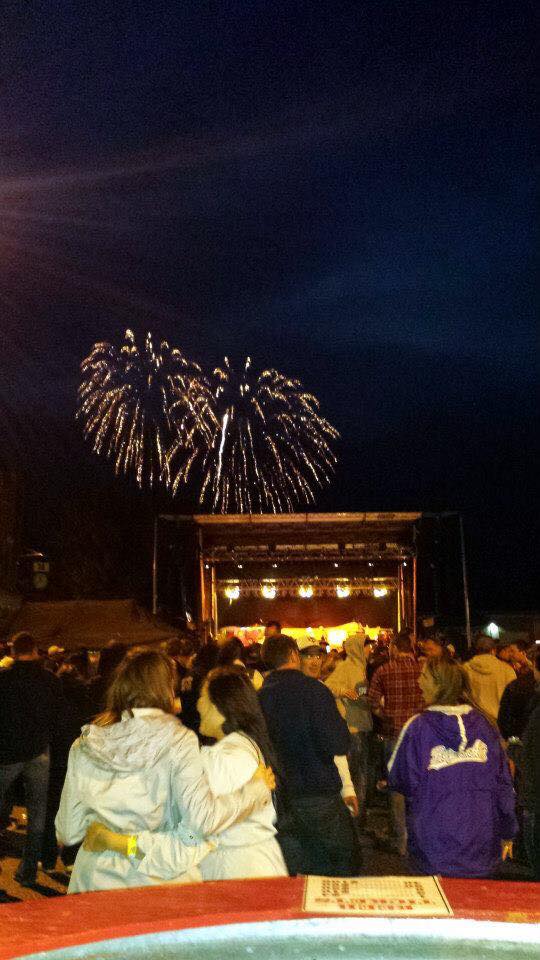This nighttime photograph captures a lively festival scene with fireworks illuminating the dark sky in the distance. The golden fireworks cascade down, framing a small, well-lit stage with five lights. It's clear that the stage is currently unoccupied, suggesting a pause in the performance. The foreground is packed with a crowd of people enjoying the event. Centered in the image are two women, both dressed in white, sharing a side hug, one wearing a yellow bracelet. They stand near a cart with a distinctive red hood that bears a logo. To the right, a woman in a purple sports jacket turns to look over, her face reflecting awe. She is next to a man dressed in dark clothing who leans slightly, engaged in conversation. The camera’s flash highlights these figures, bringing them into sharp relief against the backdrop of the vibrant festival atmosphere.